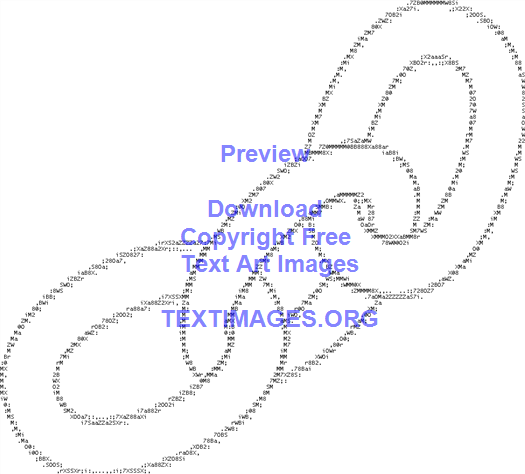The image features a white background showcasing three interlocking rings resembling chain links, created using a pixelated style typical of computer-generated text art. The rings are black on the outside and white on the inside, formed by small, indistinct numbers. The arrangement of the rings places one on the right, another centered and interlocking with both the others, and a third below. In blue capital letters above the rings, it reads "PREVIEW," followed by "download copyright-free text art images," and the website "textimages.org."